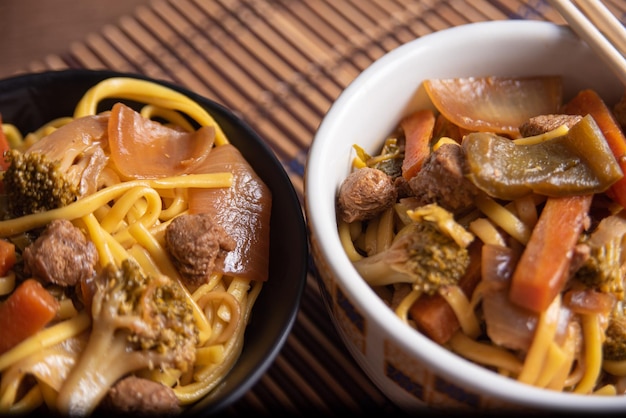This detailed photograph features two bowls of vibrant Asian cuisine artfully arranged on a wooden placemat made of interconnected bamboo pieces. The bowl on the left, which dominates the left side of the image, is black and contains a colorful array of lo mein noodles, onions, broccoli florets, beef, and long-cut carrots. To the right, a slightly larger bowl in white, adorned with red and blue patterns, mirrors the contents of the black bowl but also includes green peppers and a small mushroom. Perched on the upper right edge of the white bowl, a pair of chopsticks extends into the top portion of the photograph. The stir-fried noodles glisten enticingly, showcasing a moist and delicious appearance that enhances the overall visual appeal.